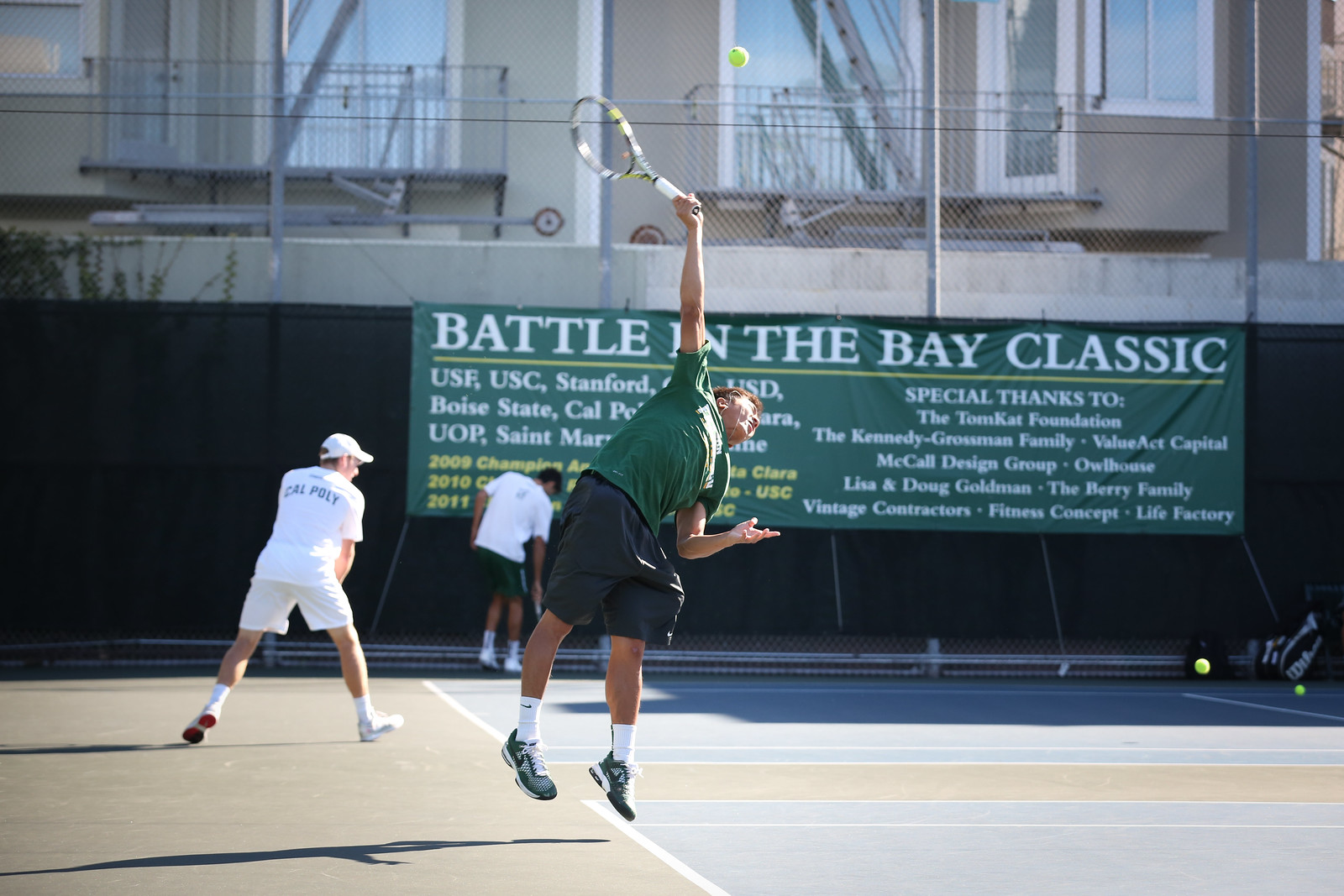In the foreground of this dynamic outdoor tennis scene, a player wearing a green t-shirt, dark shorts, white socks, and athletic shoes is captured mid-jump, extending his racket to strike a yellow tennis ball at the top of the image. The court beneath him features blue and gray rectangles with distinct white lines marking the boundaries. Behind this main player, another individual dressed in an all-white outfit, including a white baseball hat, is preparing for his turn. The scene is framed by a notable green banner on the black wall in the background, which reads "Battle in the Bay Classic" and includes acknowledgments to various foundations and sponsors. Visible beyond the court is a building with tan walls, glass doors, balconies, and multiple windows, suggesting a close proximity between the residential area and the tennis facilities.